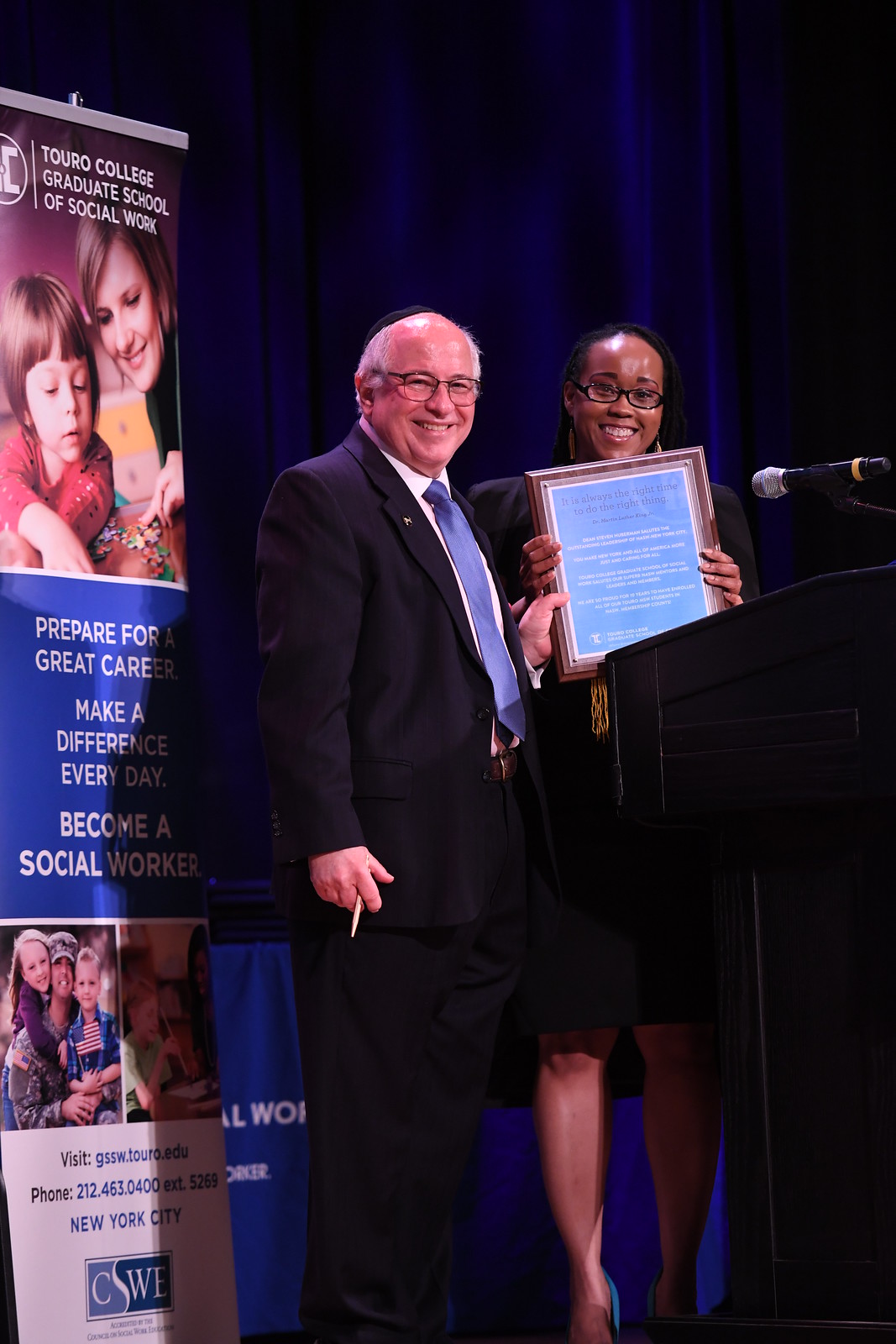The color photograph, captured in portrait orientation, showcases a stage scene set against a dark blue curtain. Central to the image are two individuals smiling and facing the camera. On the left stands an older man in a dark suit, a blue tie, and a white shirt; he has a receding hairline, white hair, and dark glasses. To his right is a young woman in a black top and skirt, also wearing dark glasses, and holding a gold-framed, blue plaque. Both are near a podium with a microphone.

A prominent sign reading "Toro College Graduate School of Social Work" is displayed on the left side of the image. Beneath this text is an illustrated photograph showing an older woman in her 30s and a little girl engaging in play, possibly making a necklace or working on a colorful toy. Below this illustration, a blue square contains the text, "Prepare for a great career, make a difference every day, become a social worker," in white font. Two additional pictures are situated below, depicting happy, smiling people who appear familial. Overall, the image conveys a welcoming atmosphere of celebration and encouragement towards a career in social work.